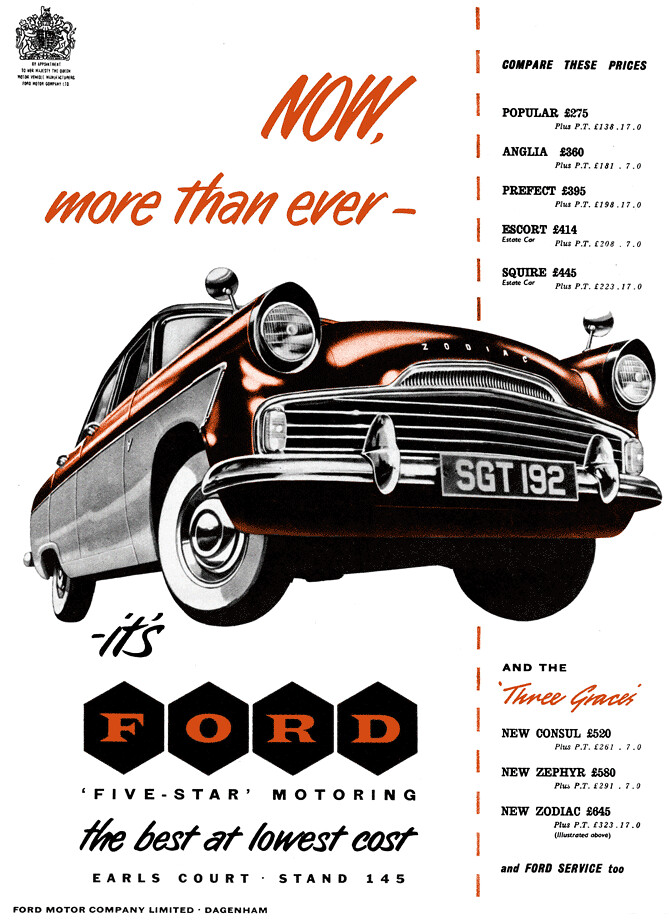The image is a detailed rendering of a vintage Ford Zodiac, presented as an advertisement for Five Star Motoring. The illustration features a burnt orange, black, and white color palette. The car, positioned centrally and facing from left to right, is labeled "Zodiac" with the license plate "SGT 192." Above the car, bold orange text reads "NOW MORE THAN EVER." Below the car, blocks in black with orange lettering spell out "F-O-R-D." Additional text beneath reveals the tagline, "Five Star Motoring - the best at lowest cost."

On the right side of the image, a list showcasing different pricing options for various models is displayed under the heading, "Compare These Prices." The prices include:
- Popular: 275 pounds
- Anglia: 360 pounds
- Prefect: 395 pounds
- Escort: 414 pounds
- Squire: 445 pounds
- Consul: 520 pounds
- Zephyr: 580 pounds

There is also mention of Ford Service, and the text "Earl's Court Stand 145" is present, indicating more promotional details. The background includes burnt orange text and black diamonds on a white backdrop, while other elements use black lettering.